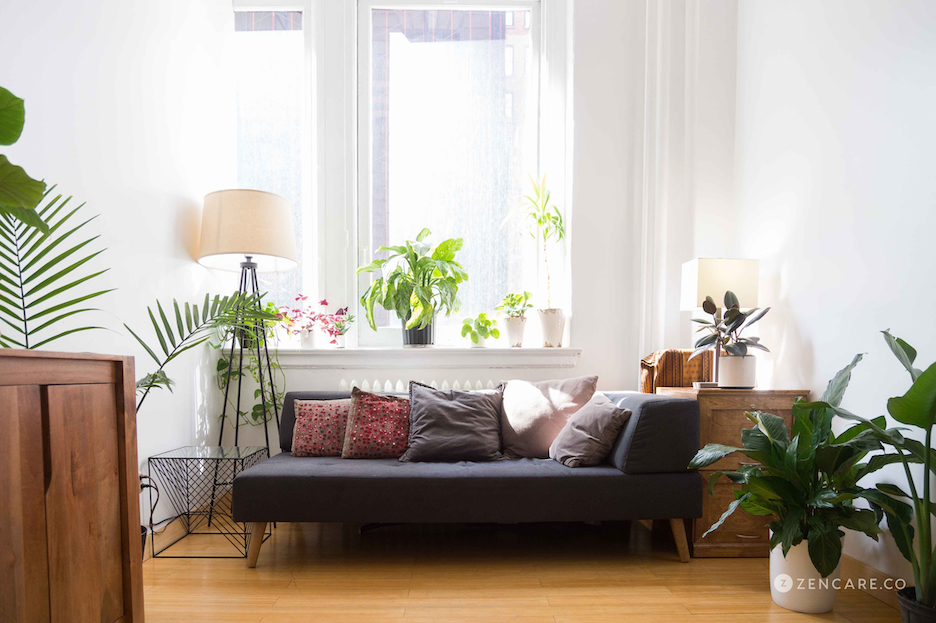The image is an advertisement for Zencare.co, portraying a serene living room with white walls and light wooden floors, warmly lit by abundant natural light streaming through a large frameless window. Central to the room is a sophisticated dark grey sofa with slanted arms and wooden legs, adorned with five assorted pillows: two black or grey, one cream, and two red with speckled patterns. Flanking the sofa, an array of greenery dots the space, with plants perched on the windowsill and scattered amongst various contemporary furnishings.

To the left of the sofa, a modern glass-topped end table, set on a black wire mesh frame, sits next to a tall floor lamp boasting a sleek white lampshade, casting gentle light over the corner. This side also features a discreet wooden chest with an intricate niche handle and a suggestive green branch hinting at another out-of-sight plant.

On the opposite side, closer to a tall window with thin white curtains, another end table displays a small green plant in a white pot and a miniature lamp, further styled by a larger potted plant with broad leaves resting on the floor.

Completing the setup, a wooden shelf houses additional decor, complementing the white and wood aesthetic that ties the room together. The clean, tranquil environment is effortlessly brightened by the interplay of white walls and ample sunlight, accentuated by the logo of Zencare.co featuring prominently in the lower right-hand corner, inviting viewers to a curated blend of simplicity and natural beauty.